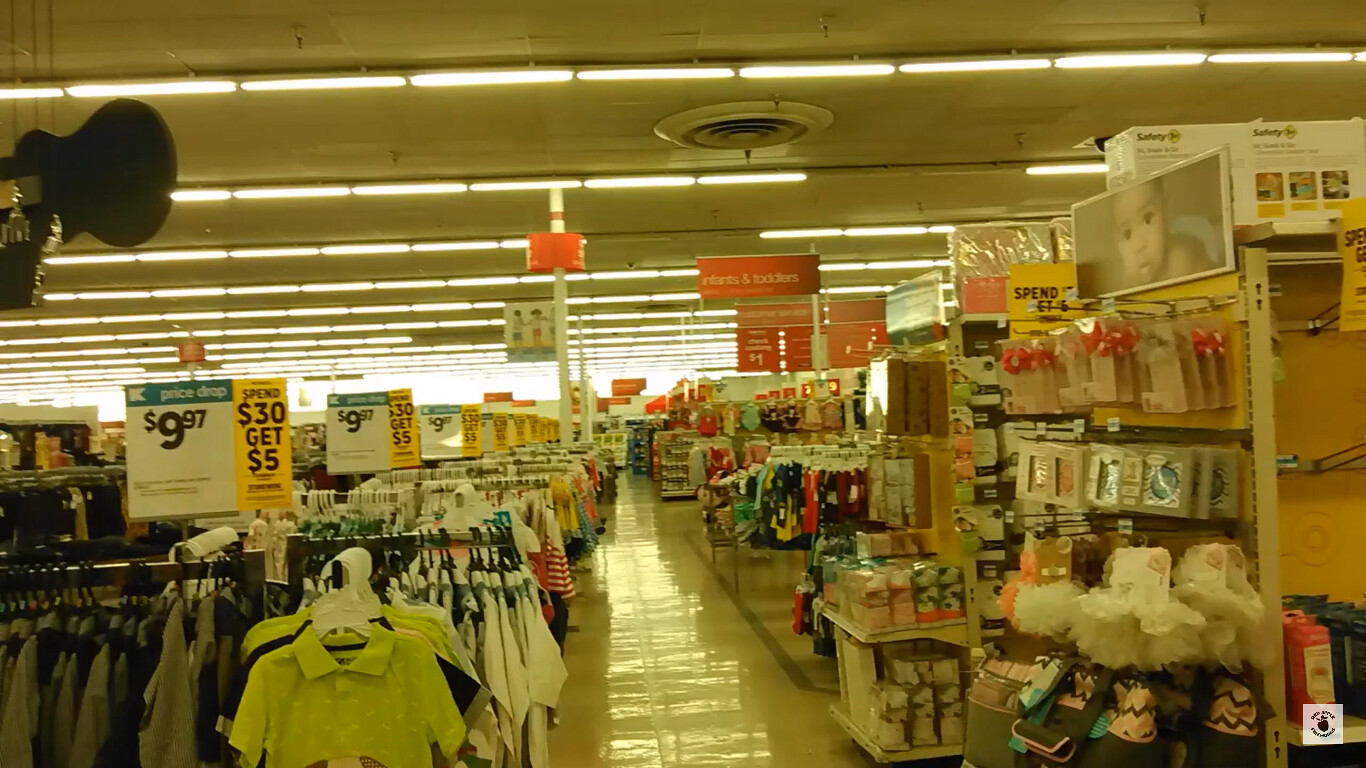This color photograph captures the interior of a department store with a gleaming white-tiled floor, reflective of the overhead fluorescent lighting. The ceiling adorned with red and white signage prominently displaying promotional offers, such as "Spend $30, Get $5” in black font on a yellow background, and "Price Drop: $9.97." The left and right sides of the image are lined with racks of baby clothing, featuring shades of green, gray, white, and striped patterns, some marked down to $9.97. In the background are more garments, possibly children's clothing in various colors including gray, burgundy, yellow, orange, and blue. Overhead, a security camera keeps watch, and a photo of a baby reinforces the focus on children’s apparel. Despite some ambiguity, this vibrant and busy retail scene is bustling with merchandise and promotional signage.